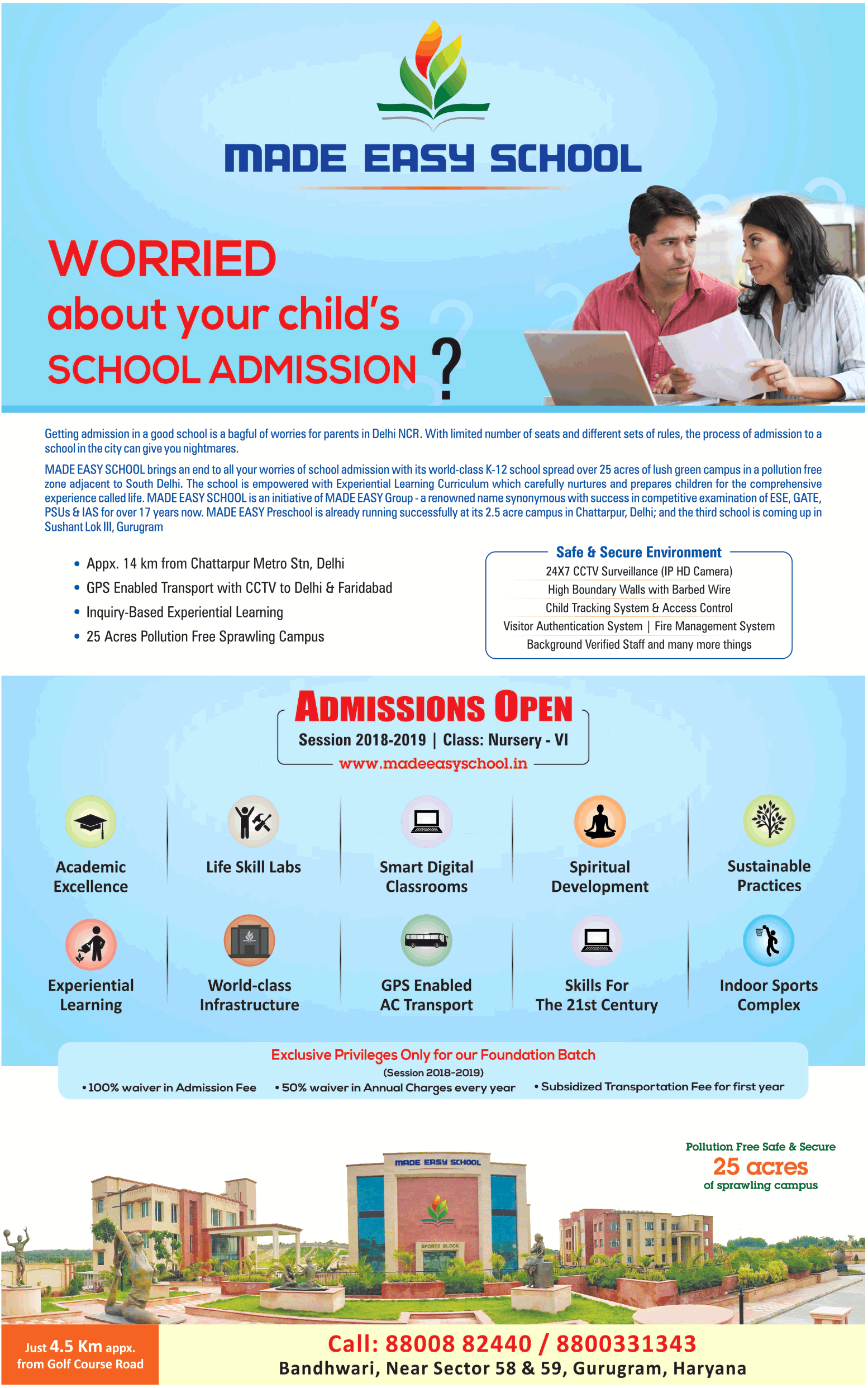Here is a cleaned-up and detailed caption for the image described:

---

The website features a prominent blue rectangle banner at the top, which stretches horizontally across the screen. In the middle of the banner, the phrase "Made Easy School" is written in blue text. Just beneath this text, an orange line accentuates the header, running only under the font on the left side.

Lower on the webpage, in red text, a message reads, "Worried about your child's school admissions?" Accompanying this message, on the right side, is an image of two parents with dark hair. The father is dressed in a red shirt, while the mother wears white. The parents are engaged in a focused conversation, with the mother holding a piece of white paper and the father viewing a laptop, the back of which is visible to the viewer.

Below these visuals, a paragraph of small print explains the challenges of school admissions in Delhi NCR. It speaks to the limited number of seats and varying regulations that make the admissions process stressful for parents. The content highlights that "Made Easy School" alleviates these concerns with its world-class K through 12 education on a sprawling 25-acre, green, pollution-free campus adjacent to South Delhi. The school is distinguished by its experiential learning curriculum, designed to thoroughly prepare children for life.

"Made Easy School" is a venture by the Made Easy Group, a well-known name synonymous with success in competitive examinations such as ESE and GATE.

---